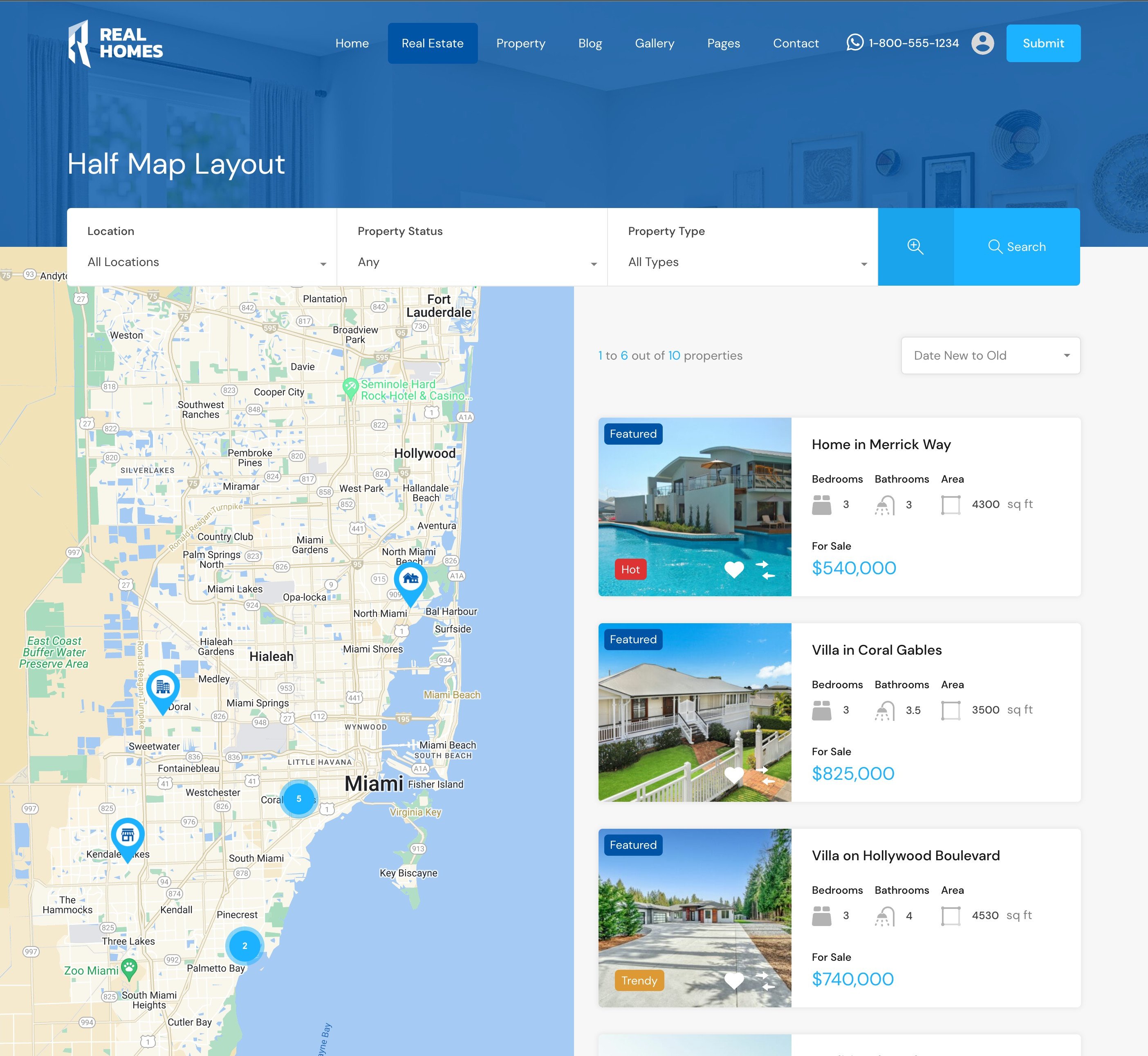At the top, a blue border features the title "Real Homes", alongside clickable navigation options such as Home, Real Estate, Property, Blog, Gallery, Pages, and Contact. A phone icon displays the number 1-800-999-1234. Below this, the header "Half Map Layouts" appears, accompanied by a drop-down menu box labeled "Location", defaulting to "All Locations". Additional drop-downs include "Property Status" set to "Any" and "Property Type" set to "All Types". To the right, there are two search buttons: a standard one and another featuring a magnifying glass icon labeled "Search".

On the left side, a detailed map of Miami is displayed, marked with five blue location pins scattered across various areas. To the right of the map, three thumbnail images showcase different homes, with one prominently labeled "Home Merit Way" and listed for sale at $540,000.